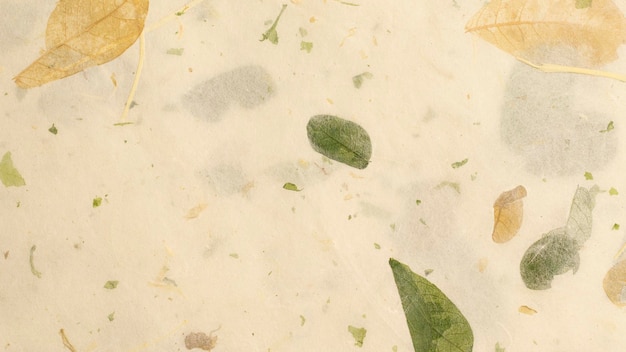This image is a rectangular watercolor painting, longer from left to right than it is from top to bottom, featuring a subtly pinkish white background. It is adorned with an array of leaves and organic fragments. Speckles of green, cream, orange, and yellow are scattered throughout the composition, imparting a delicate, almost speckled texture to the piece. 

In the top right corner, there is a leaf resembling that of a ficus benjamina, very faded, giving it a rotted look. The bottom left contains a sharply defined, gray-green leaf suggestive of eucalyptus, and directly above it, another leaf mirrors this style but appears more rounded. The middle of the painting hosts a forest green leaf without a visible stem. To the bottom center, there’s a wide-based leaf tapering to a tip, and nearby, a curled orange leaf accompanied by another green one.

Additionally, some leaves seem broken or fragmented, with chips of leaves and branches sprinkled across the page, enhancing the sense of depth and dimension. Shadows cast by some elements, shown in darker gray areas, contribute to an illusion akin to looking at leaves underwater. Despite their faded and delicate appearance, these leaves offer intricate details, such as visible veins on the orange-hued leaf in the left corner, anchored by a white stem, creating a rich tapestry of colors and layers.